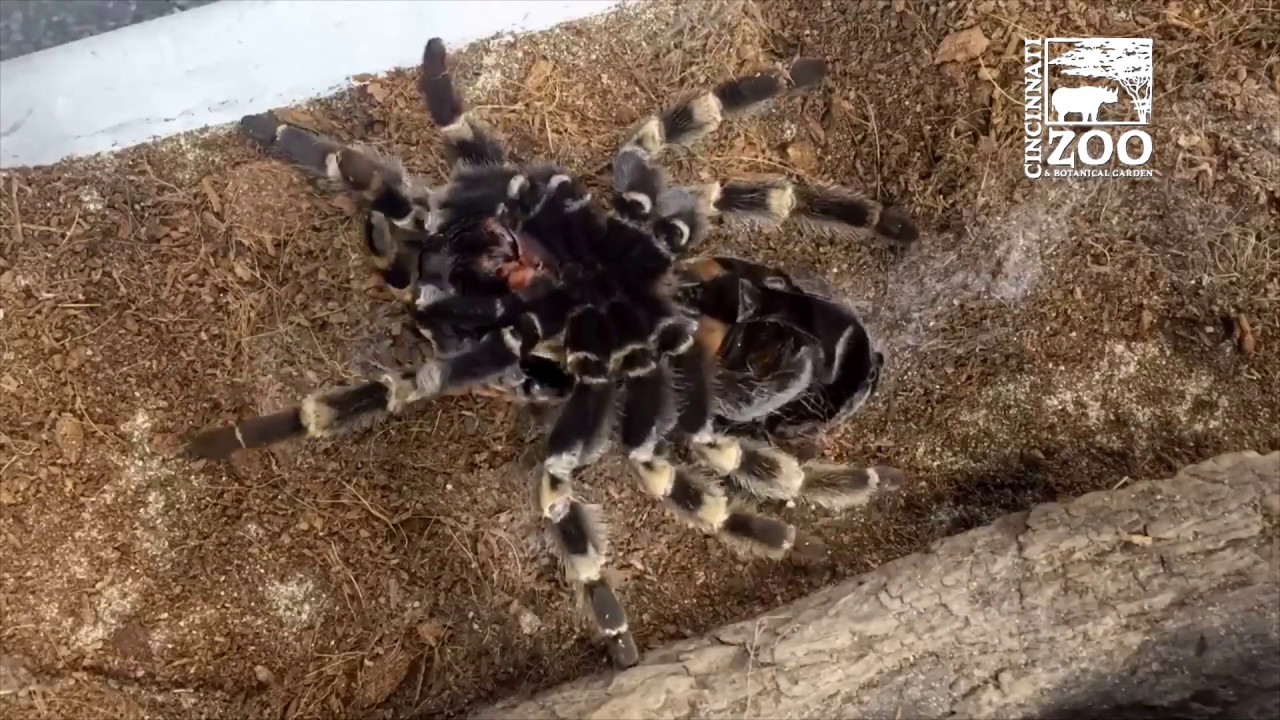In this close-up image, a large tarantula is prominently displayed, occupying the entire frame. The tarantula's body is primarily black with segments of tan, brown, and occasional shades of reddish-orange, particularly noticeable on its upper body. Its legs are covered in a mixture of black and tan hairy fur, adding texture and detail. Beneath the spider, the terrain includes pieces of dirt, crumpled leaves, small twigs, brown moss, and a light brown log, suggesting a naturalistic enclosure. The top right corner of the image features the Cincinnati Zoo's logo, which includes a white silhouette of a rhinoceros standing under a tree, accompanied by the text "Cincinnati Zoo & Botanical Garden."